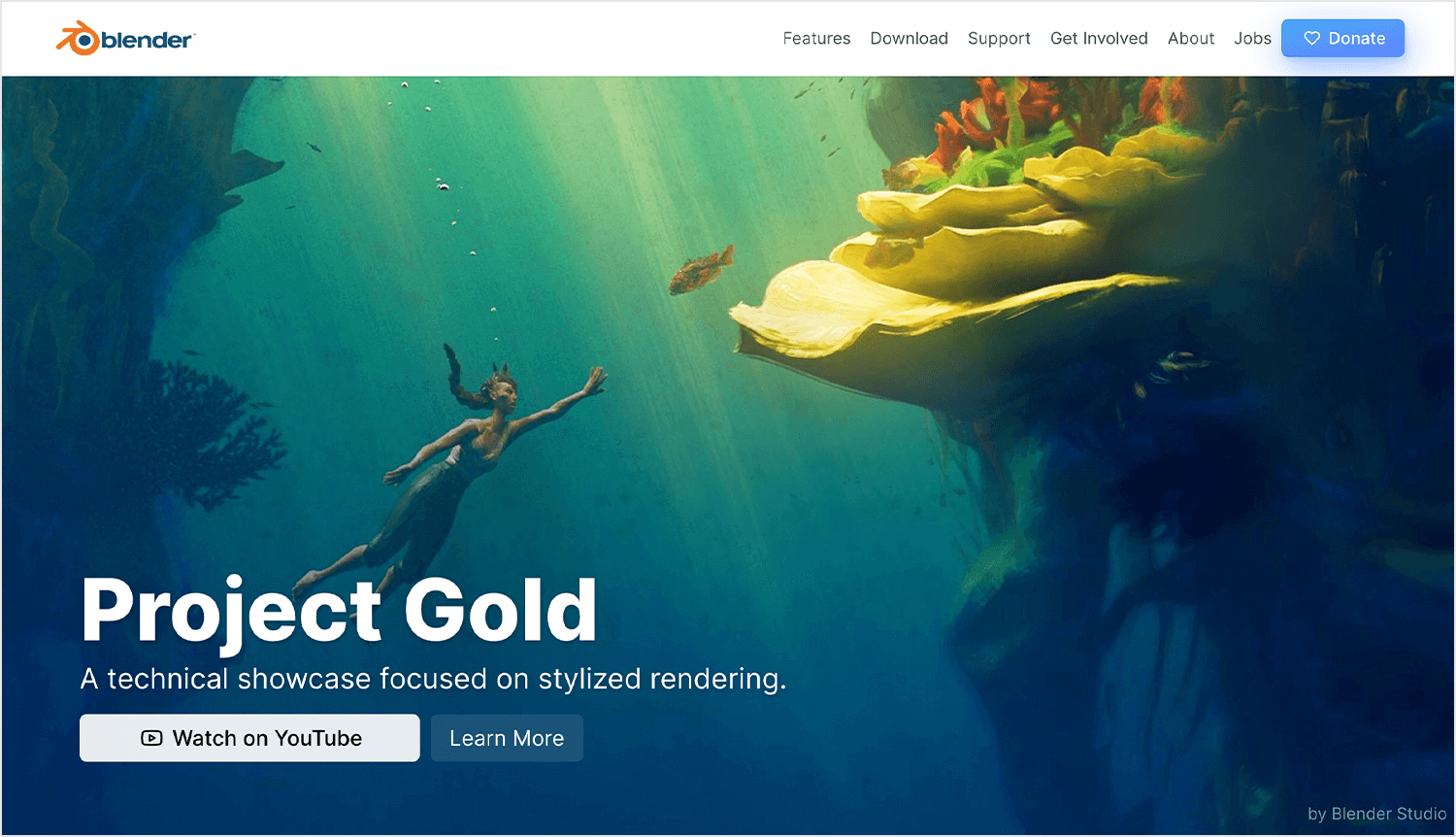Here's the revised and detailed caption:

---

This screenshot captures the homepage of a website. Dominating the screen is a large photograph that occupies approximately 80% of the space. The top of the page is adorned with a clean, white navigation bar. In the top-left corner, there's a distinctive logo: an orange circle with three extending lines, reminiscent of a cockerel's comb, featuring a central blue dot. Adjacent to the logo, the website name "Blender" is written in dark blue lowercase letters.

The navigation bar includes several options: "Features," "Download," "Support," "Get Involved," "About," "Jobs" (marked by a blue dot above it), and "Store." In the top-right corner, there is a light blue button with a white heart icon and the word "Donate."

The prominent image appears to be an imaginative nature scene. It showcases various plants, and centrally, an adult creature accompanied by two baby creatures. These fantastical beings are white and brown, with striped tails and beak-like features, clearly products of creative design rather than real-life animals.

Positioned centrally and left-justified within the image is a bold, multi-color text against a black background: "Blender 2.92 is out!" The text starts with yellow at the "B" and transitions to pink at the exclamation point. Directly below this, another black block contains text promoting the new version: "A completely new workflow for editing meshes, new physics simulation methods, and so much more." This message also transitions from yellow to pink.

Beneath this central image, in white text, the site declares: "Open source 3D creation, free to use for any purpose forever." Adjacent to this statement, a blue block with white text invites users to "Download Blender 2.92.0."

---

This detailed caption encapsulates both the visual and textual elements of the screenshot, providing a comprehensive description.